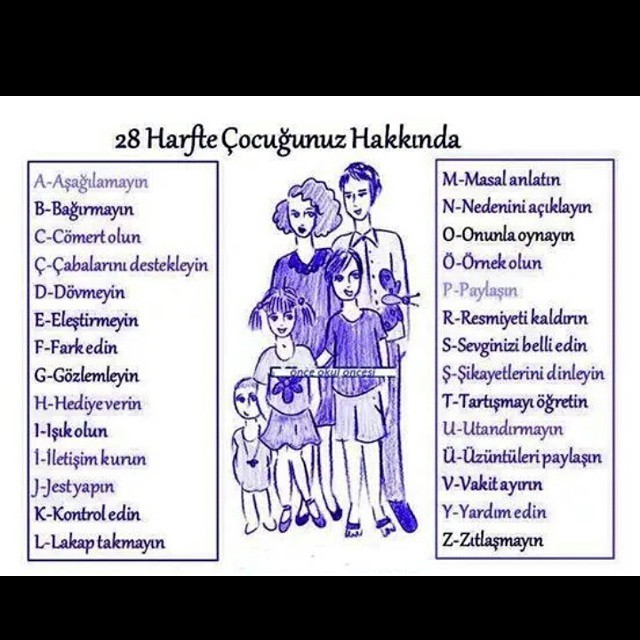The image is of a family portrait drawn in blue ink or purple pencil, featuring a mother, a father, and three children—a young boy, a young girl, and a toddler whose gender is indeterminate. The mother, positioned on the left, has bushy, blonde hair and is wearing a purple dress. The father stands on the right, also dressed in purple. The young boy, in front of the father, and the young girl, in front of the mother, are wearing light purple. In between the mother and the young girl is a toddler who is also part of the family.

The poster background is predominantly white with thick black bands along the top and bottom edges. At the top of the image is a bold black title featuring the number "28", followed by words written in a foreign language that organize the alphabet alongside corresponding words. On the left side, the words are listed in alphabetical order from A through L, while the right side continues from M through Z. Each side has these words outlined in black rectangle boxes. Above the family, there appears to be a butterfly, adding a whimsical touch to this illustrative image possibly taken from a children's book.